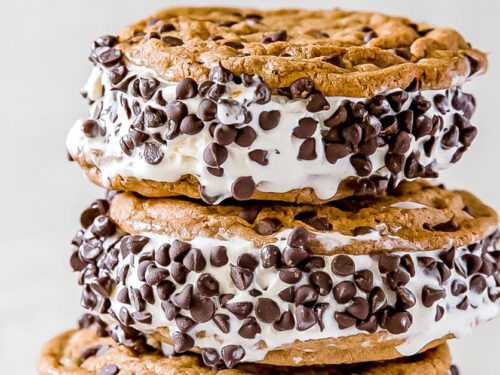This close-up photograph captures a stack of delectable ice cream sandwiches against a light grey background. At the base, we can see the upper part of a golden brown chocolate chip cookie. Resting on it, slightly shifted to the right, is a sandwich formed by two deliciously golden chocolate chip cookies embracing a thick, two-centimeter band of creamy vanilla ice cream. The ice cream's exterior is adorned with mini chocolate chips, adding texture and visual appeal. Another identical sandwich sits on top, slightly offset to the left, following the same pattern with melting ice cream trickling around the edges. Despite the slight cut-off at the bottom of the image, the detailed textures of the stacked, irregularly aligned cookies with their rich chocolate chips and creamy vanilla ice cream are clearly highlighted.